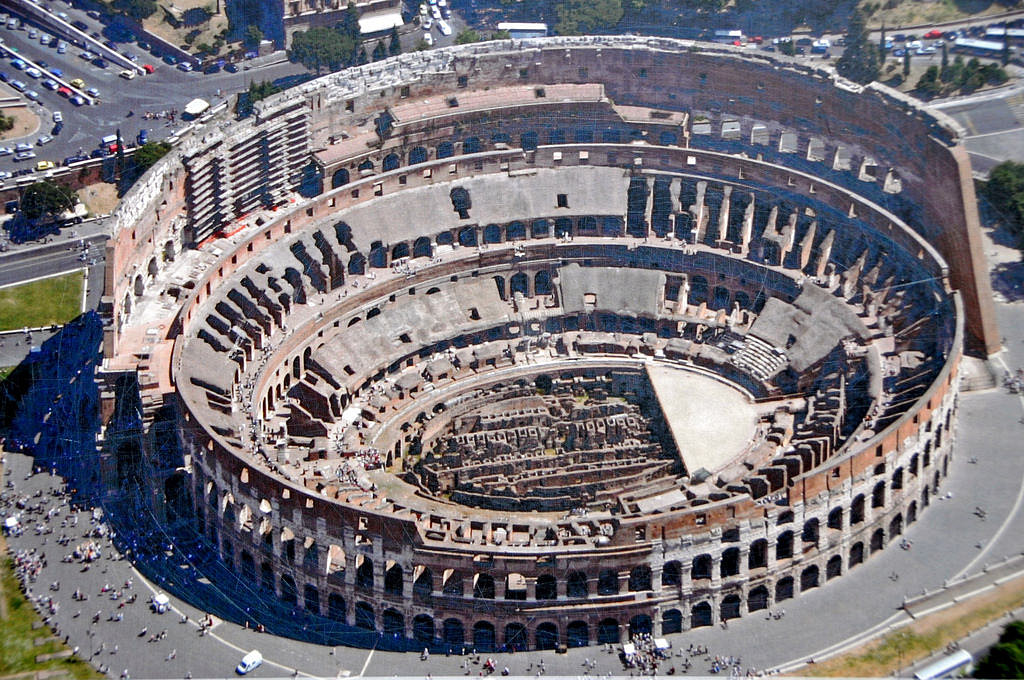This aerial photograph, taken on a bright, sunny day, depicts the ancient Colosseum in Rome from a high vantage point, likely from a helicopter or drone. The angle of the shot provides a comprehensive view into the decayed structure, revealing multiple levels including the labyrinth-like center, the semicircular partial stage on the right-hand side, and the pit. The ruins display various sections of broken and dilapidated walls in shades of grey and brown. The grand, oval-shaped coliseum features multiple tiers, with the back being the tallest segment and the front adorned with two rows of arches encircling the edges. Scattered around the exterior are tiny, ant-like people, suggesting a heavy tourist presence, and a ring road with minimal traffic implying restricted vehicle access. Surrounding the historic site, modern Rome is clearly visible with busy highways packed with cars and scattered greenery including hedges and trees.